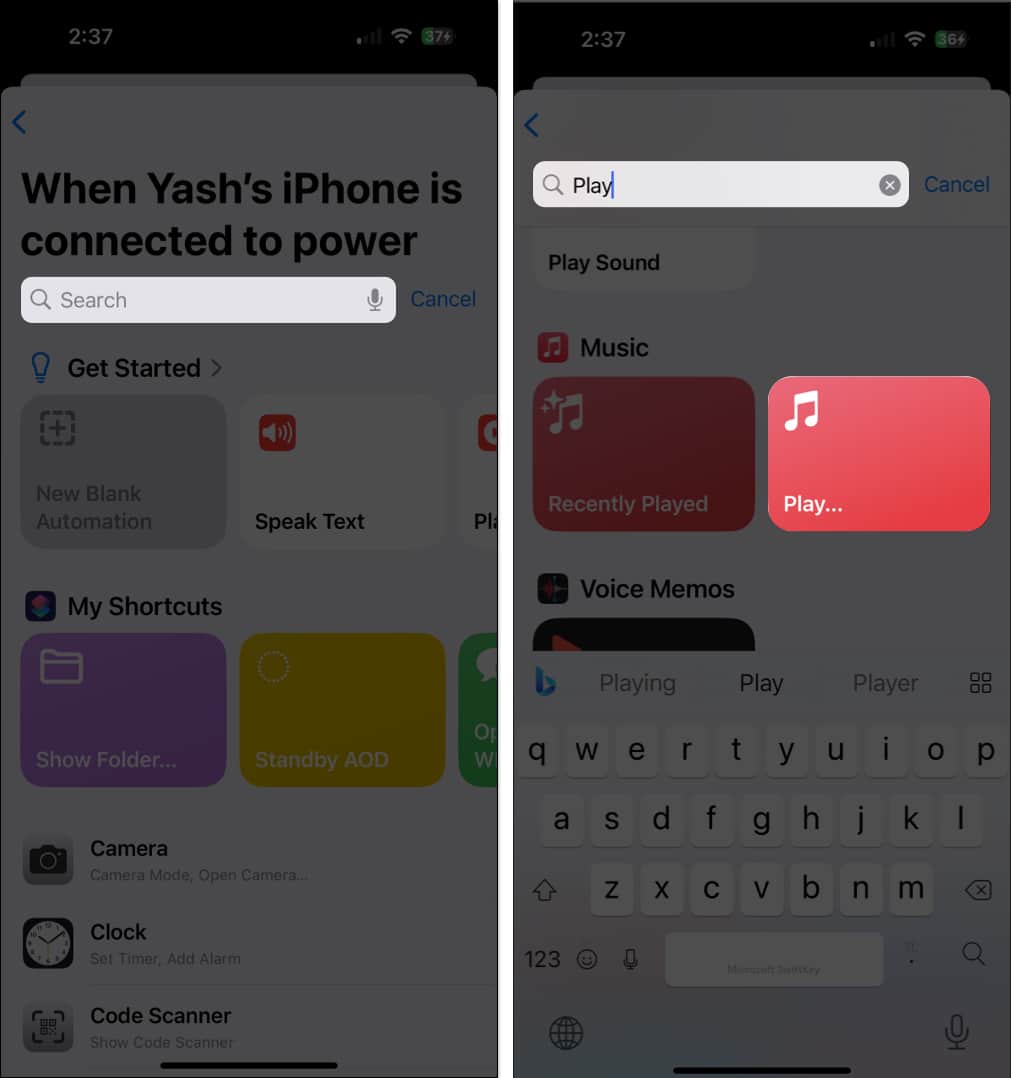Here is the cleaned-up and detailed caption for the image:

"In this image, we see two cell phone screens side by side, each displaying a holographic gray background. 

The left screen shows the following details from top to bottom:
- At the top-left corner, the time is displayed as '2:37', with the battery percentage and Wi-Fi signal icons to its right.
- Below, it states 'Yash's iPhone is connected to power' with a search bar underneath.
- Further down, the text reads 'Get Started' followed by three square icons:
   - The first square is labeled 'My Shortcuts' in purple, indicating a folder.
   - To its right, the second square is labeled 'Standby' in green.
   - Below these, visible partially, is an icon for the 'Camera', 'Clock', and 'Code Scanner'.

The right screen displays:
- The search bar is actively being used, with the word 'play' being typed out.
- Below the search bar, options listed are 'Play Sound' and 'Music'.
- A red square labeled 'Recently Played'.
- Below that, a highlighted pink square labeled 'Play...'.
- Then 'Voice Memos' is listed.
- We see about 20% of a black square featuring a pink triangle icon.
- The bottom portion shows a keyboard with a gray background; the letters are black and the keys are white.

This detailed layout forms the complete interface depicted on both phone screens from top to bottom."